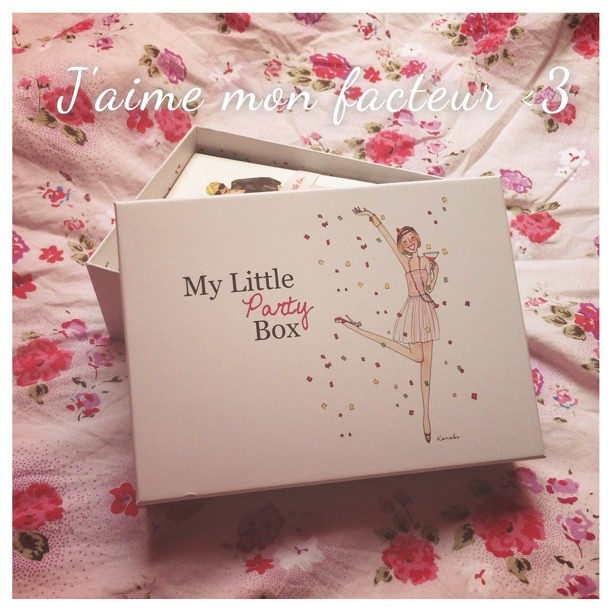The image showcases a white gift box titled "My Little Party Box," placed open on a predominantly white bed adorned with red roses and floating petals. The box lid, slanted against the main body, faces the viewer and features an illustration of a joyful woman in a short skirt and dress, one leg playfully raised, scattering flower petals. The text "Party" is written in cursive red, while the remaining text is in black. Above the box, there is French text reading "J'aime mon Facteur," followed by "S3." Inside the box, partially visible, is a white sheet of paper displaying the face of a blonde woman wearing sunglasses and a black shirt, suggesting the contents are a part of the box's theme of celebration and enjoyment. The overall scene is set against a floral bedspread, enhancing the festive and lively atmosphere.